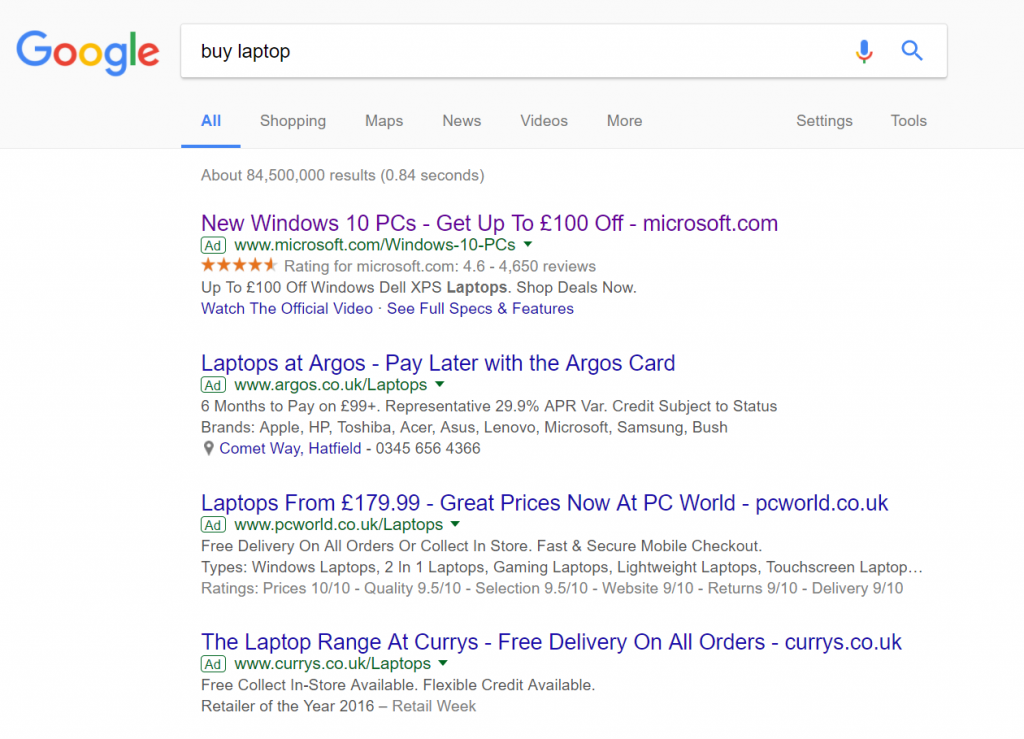A Google search for "buy laptop" is displayed on a laptop screen. The search bar at the top includes a microphone icon and a search icon. Above the search results, various menu tabs are visible, including "All," "Shopping," "Maps," "News," "Videos," and "More," with "Settings" and "Tools" to the right.

The search returned approximately 584,500,000 results in 0.84 seconds. The top result, marked as an ad and clicked on, is for "New Windows 10 PC" from Microsoft, offering discounts up to €100. Below this, there are three additional ads: "Laptops at Argos - Pay Later with the Argos Card," "Laptops from €179.99 - Great Prices at PC World," and "Laptop Range at Curry's - Free Delivery on All Orders." Each result includes a brief description and the store's website, emphasizing the commercial nature of the search results.